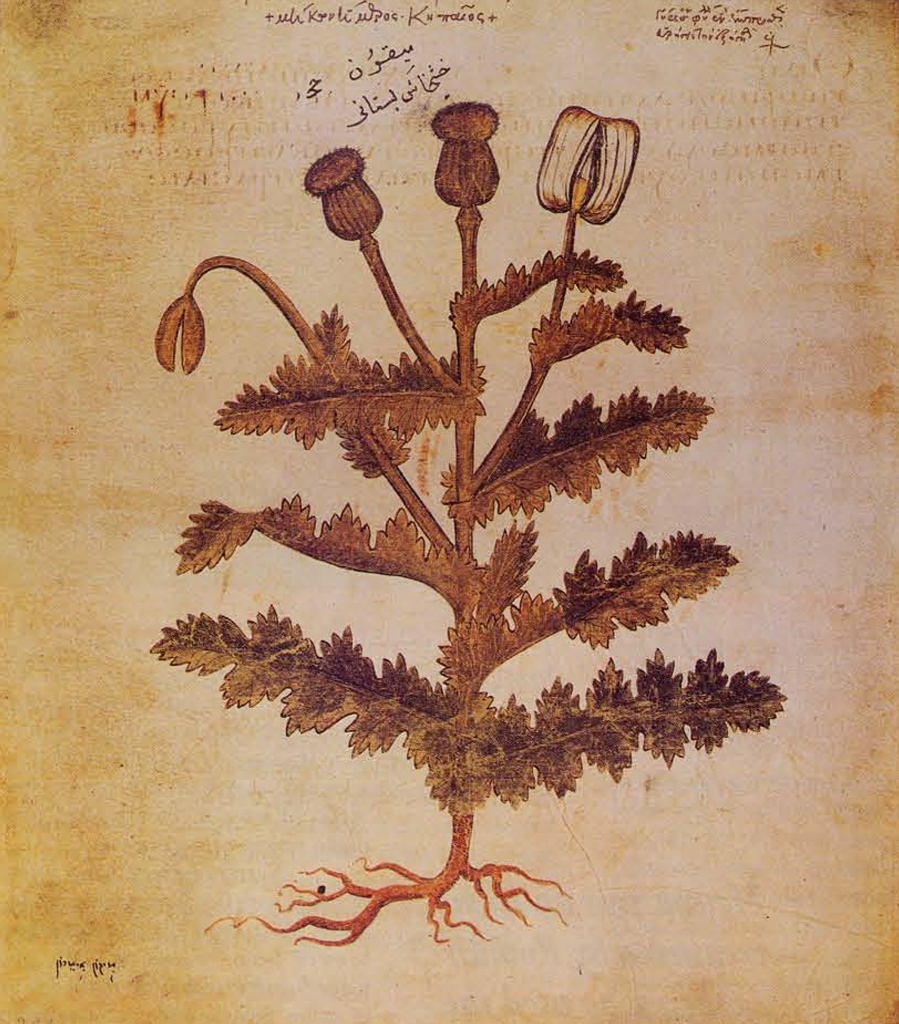This detailed caption incorporates elements from each person's description, with an emphasis on shared and repeated details for clarity and depth:

"This illustration, appearing to be hand-drawn and possibly from an old book, depicts a bush with intricate detail. The roots are illustrated in brown, sprawling in different directions, supporting a single main stem that rises prominently. The stem branches out into three rows of green leaves, with some leaves appearing empty or peeled, akin to a dandelion stripped of its petals. Among the foliage, there are various stages of flowers; two smaller closed buds near the top, a drooping flower on the left showing only its center, and a single flower on the right with a yellow center and partially closed white petals. The background canvas has a weathered, antique look, with umber smudges around the edges, enhancing its aged appearance. At the top of the image, there is text in a foreign script, possibly Arabic or South Asian, while a faint illustrator's signature is visible in the bottom left corner. The illustration serves as an identification guide, displaying the plant's roots, stem, leaves, and buds in various blooming stages, rendered in shades of brown, sienna, and umber."